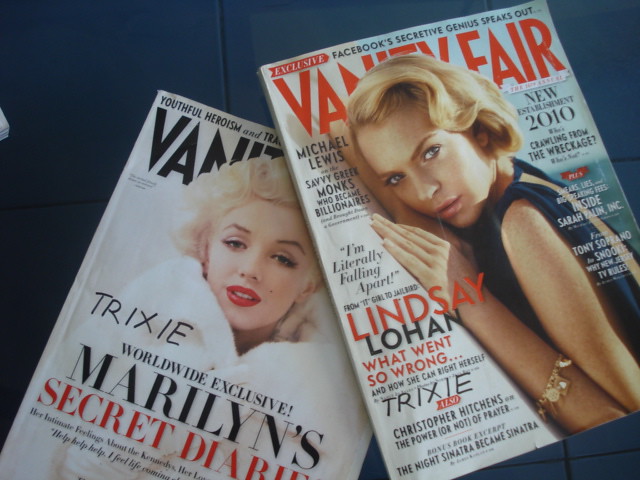Two Vanity Fair magazines are displayed on a dark navy blue surface. The magazine on top features a red Vanity Fair title and highlights various articles, including "Exclusive: Facebook’s Secretive Genius Speaks Out" and "Lindsay Lohan: What Went So Wrong?" The cover photo is of Lindsay Lohan lying on what appears to be a white background, possibly a bed or beach, with her blonde hair styled in short curls reminiscent of Marilyn Monroe, wearing a blue dress and looking directly at the camera. Additional articles mentioned include "Michael Lewis: Savvy Greek Monks Who Became Billionaires" and "Christopher Hitchens: The Power or Not of Prayer."

The second magazine, partially obscured by the first, has a black Vanity Fair title. It features an exclusive on "Marilyn's Secret Diary" with the headline "Worldwide Exclusive: Marilyn's Secret Diaries," alongside a photo of Marilyn Monroe wrapped in a white bathrobe and wearing bright red lipstick. The cover teases intimate details about her feelings towards the Kennedys, and a sensational excerpt at the bottom states "Help, Help, Help I Feel Life Coming." Both covers include the name "Trixie," further connecting the themes.